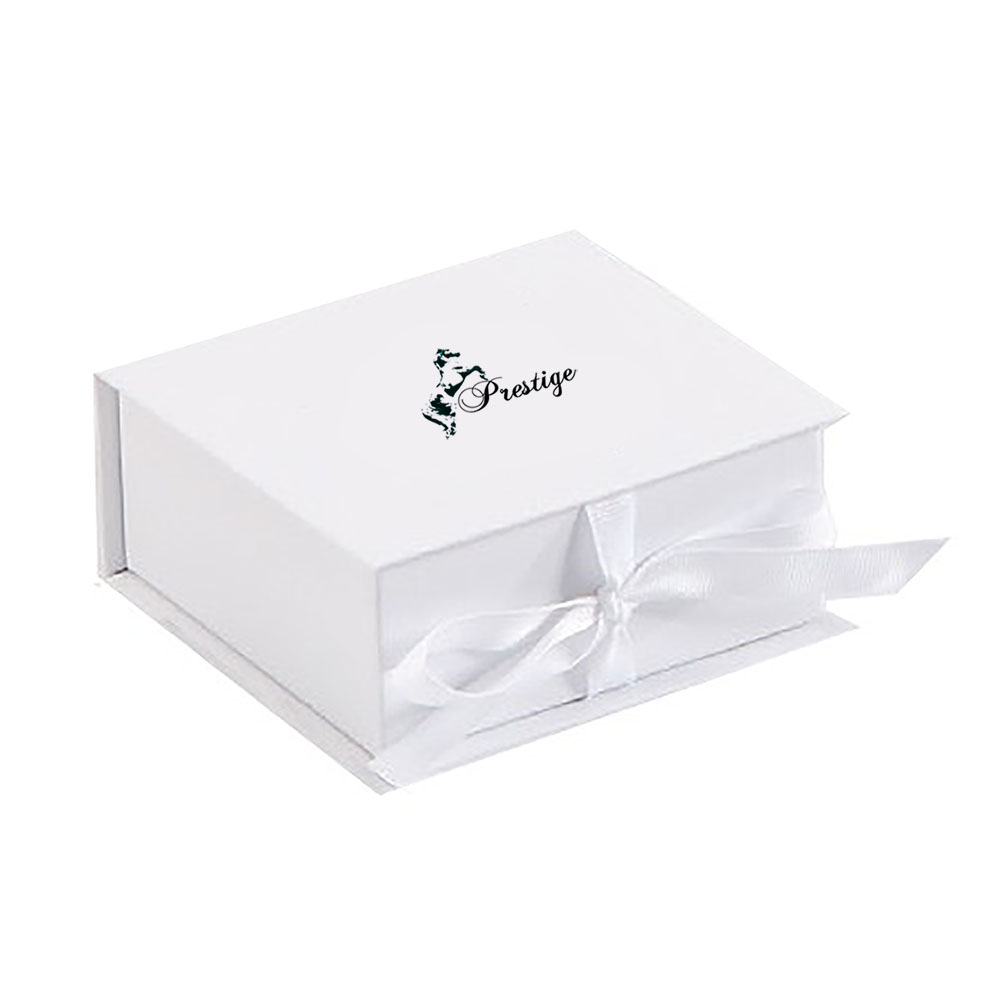The image depicts a sleek, rectangular gift box set against a plain white background. The box, crafted from a sturdy, thick material, is predominantly white and features a neatly tied white ribbon bow on its top lid, which is currently closed. The box is presented at an angle, with its top right-hand corner elevated. On the front lid, there's a sophisticated black illustration of a rearing horse, showcasing intricate detailing with shadowed elements to give it form. Adjacent to the horse, in elegant black cursive, is the word "Prestige," with the initial "P" cleverly positioned beneath the horse's hooves. The combined elements of the fancy calligraphy and the dynamic horse image create a refined and luxurious presentation.